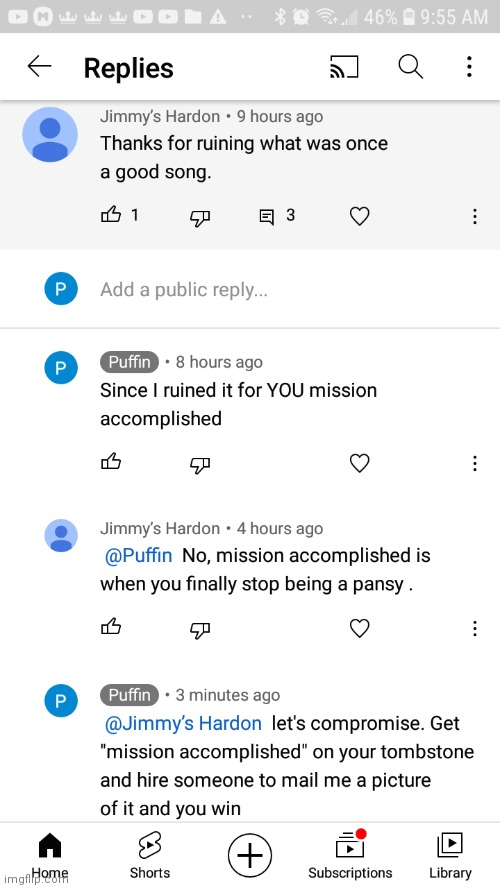**Descriptive Caption for a Screenshot of the App Interface:**

The image is a screenshot of a mobile app with a vertically oriented layout, making the display taller than it is wide. At the very top, there's a gray border populated with various icons representing different functionalities and settings of the device. In the top right corner, a timestamp reads "9:55 a.m." followed by a battery icon indicating 46% charge remaining, along with connectivity indicators for cellular signal, Wi-Fi, and Bluetooth.

On the left side of the top border, there are several more icons, including ones resembling video playback buttons characterized by rectangular shapes with triangles in the middle. Below this top section, a header labeled "Replies" indicates that the current view pertains to the replies or comment section of the app. An accompanying back arrow icon suggests an option to return to the previous page, while a search bar allows users to search within the section. At the far right end of this header is a three-dot menu for accessing additional settings or options.

The main content area is populated with user comments, each featuring a small profile image or avatar on the left. The first comment displays a default blue avatar with a generic person illustration. This comment is authored by "Jimmy’s Hardened" and was posted nine hours ago, and it reads, "Thanks for ruining what was once a good song." Another comment, seemingly a reply, says, "Since I ruined it for you, mission accomplished," featuring an avatar with a "P" next to it.

Additional comments are similarly formatted, each with a profile image, username, timestamp, and the comment text. At the very bottom of the screen, there's a navigation bar with buttons labeled "Home," "Shorts," a plus sign, "Subscriptions," and "Library," reminiscent of a layout often seen in apps like YouTube, though the specific app is not explicitly mentioned in the screenshot.